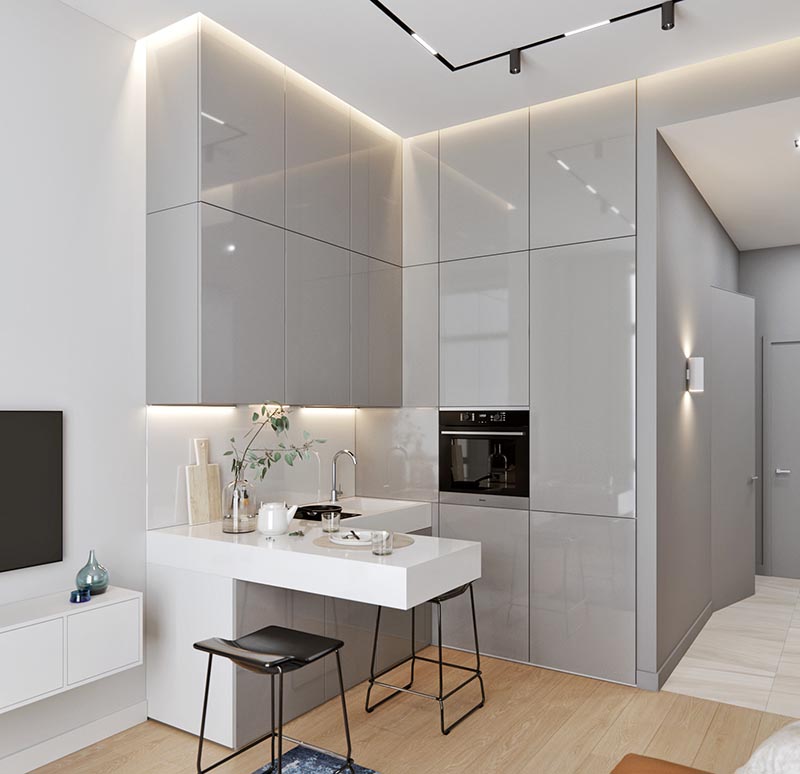In this detailed image of a very modern and luxurious indoor sitting area, the design features a sleek, modernistic kitchen. The space appears almost square in shape, with polished surfaces that exude an air of sophistication and expense. The primary color palette includes whites, grays, and silvers, creating a seamless, elegant look. Upon entering through a foyer clad in burnished silver plates, you are greeted by a white marble floor that transitions into a tan hardwood floor as you step into the kitchen—a space softened by an orange rug and a navy blue rug.

Marble surfaces dominate the room, highlighting a white island equipped with a sink, adorned with some plates, a white teapot, and a glass vase holding greenery. The cabinetry, strikingly modern and handle-less, combines high-set units with a sleek, polished silver finish. The refrigerator is hidden within these cabinets, with only the water dispenser subtly indicating its presence. There is a flat-screen TV mounted on the wall, partially cut off to the left, and adjacent to it is a small cabinet displaying green glassware.

Adding to the modern aesthetic, two wire-frame stools without back support are positioned at the island. The walls feature square and rectangular designs, further enhancing the room's contemporary feel. A black box, potentially a compact oven, is mounted on the wall. Dirty dishes sit atop the counter, reinforcing the room's function as a kitchen. The overall lighting is ample, illuminating the white, gray, and shiny surfaces beautifully, making it a very well-lit space.